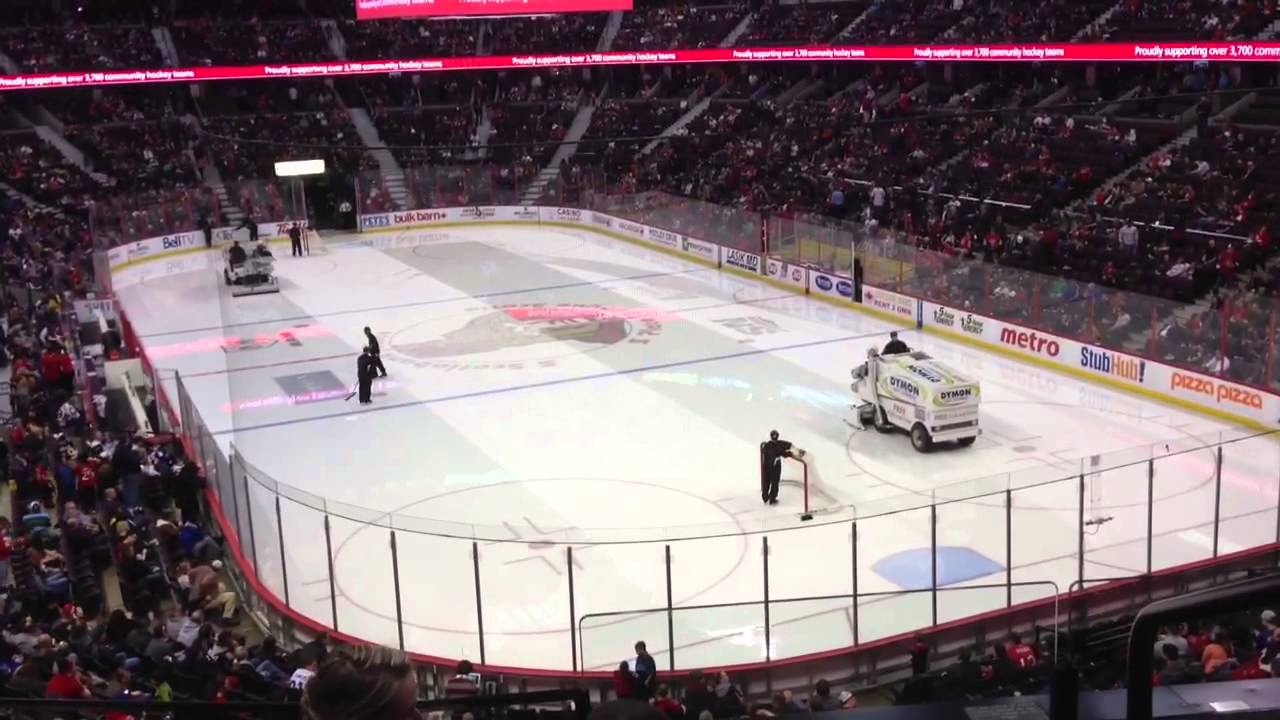The image depicts a vast, bustling ice hockey arena viewed from a second-deck seat positioned behind and slightly to the left of one of the goals. It's intermission time, and the scene is a flurry of activity with two white Zambonis smoothing the bright, white ice while a few people skate or walk behind them, using brooms or equipment to clear debris. The ice goals have been removed, and the doors where the Zambonis entered are visible in the distance. The surrounding stadium is packed with spectators, their seats arranged in multiple tiers that ascend dramatically. Staircases are interspersed between sections of seating. A prominent pink ticker tape runs around the upper deck with white lettering advertising various products and services. The framework surrounding the rink includes a high fence that rises in the corners and remains tall behind the goals, ensuring safety for the spectators in the lower rows closest to the action. Amidst the lively crowd, the intricate preparations to make the ice pristine remind viewers of the meticulous efforts that go into maintaining the beloved sport.